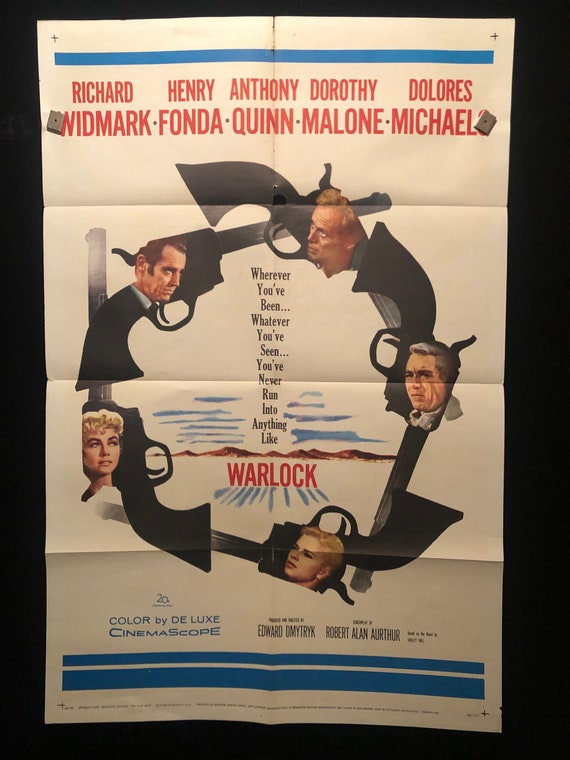The image depicts a framed movie poster for the film "Warlock," prominently featuring the names of the stars Richard Widmark, Henry Fonda, Anthony Quinn, Dorothy Malone, and Dolores Michaels written in bold red text across the top. Dominating the center is an artistic arrangement where six black revolvers form a full circle, with headshot profiles of the actors appearing within the revolver chambers. A white background enhances the clarity of the visuals, while additional descriptive text in varying hues of blue, black, and red reads: "Wherever you've been, whatever you've seen, you've never run into anything like Warlock." Below this tagline, set against a backdrop of desert-like mountains, more detailed but less legible writing appears. The left side of the poster includes text that reads "Color by Deluxe Cinemascope," and at the bottom, two blue bars are accompanied by harder-to-read black writing identifying Robert Alan Arthur and Edward Dmytryk.